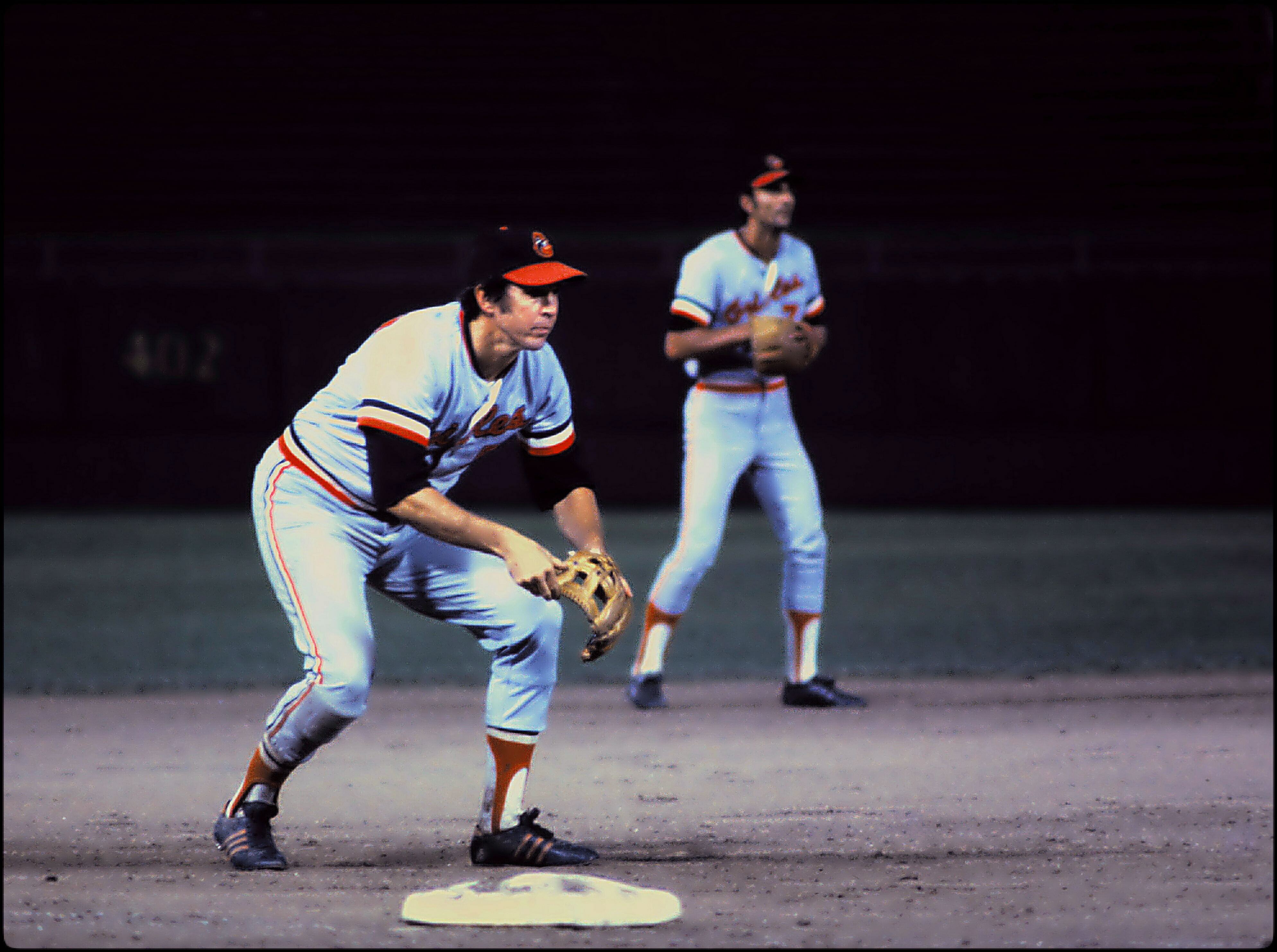The photograph captures an intense moment during a baseball game featuring former Baltimore Oriole players, Brooks Robinson and Mark Belanger. Brooks Robinson, who is positioned prominently on the left side of the image, is intently crouching near a base, ready to react to the play unfolding before him. He wears a grey uniform accented with black, white, and orange details, typical of the Orioles' team colors, along with a dark blue and red cap. With his left hand gripping his baseball glove and his right hand subtly holding its edge, Robinson epitomizes readiness and focus. Behind him, slightly out of focus yet clearly visible, stands Mark Belanger, the team's shortstop. He mirrors Robinson's poised stance, holding his glove close to his chest, prepared for any potential action. The ground beneath them is a greyish dirt infield, and the dark, indistinct background only highlights the players' alert postures. The image hints at an old-school scoreboard or wall, possibly displaying numbers like "402," but these details remain blurred and ambiguous.